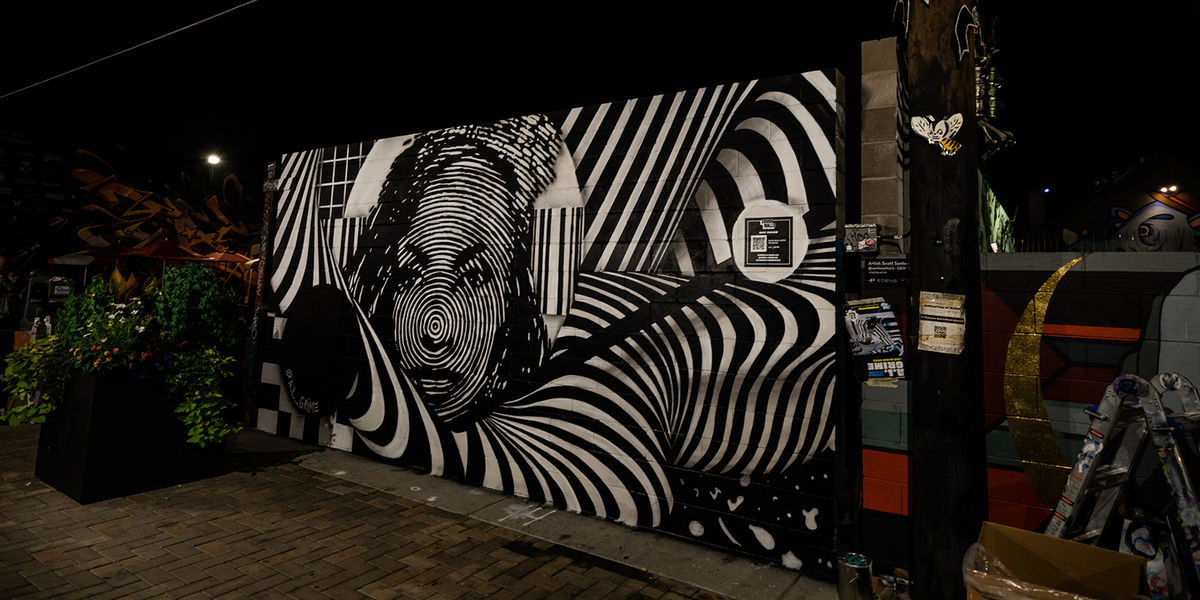The photograph captures a striking mural painted on an exterior wall, depicting a vivid, artistic zebra-like design with a woman's face at its center. The face, rendered in black and white concentric circles originating from her nose, gives a hypnotic, bullseye effect. Her black hair and lips stand out amidst the elaborate zebra stripes that extend across the mural. The background of the mural also features zebra stripes, contributing to the cohesive and surreal aesthetic. On the left side of the image, there's a planter box containing green foliage and a few orange and white flowers. The mural seems to be set against the backdrop of a black night sky, with a red brick path visible at the base of the wall. Additional details include a window framed with zebra-striped curtains, which enhance the overall intricate design. The scene blends elements of fantasy and reality, producing a mesmerizing visual experience.